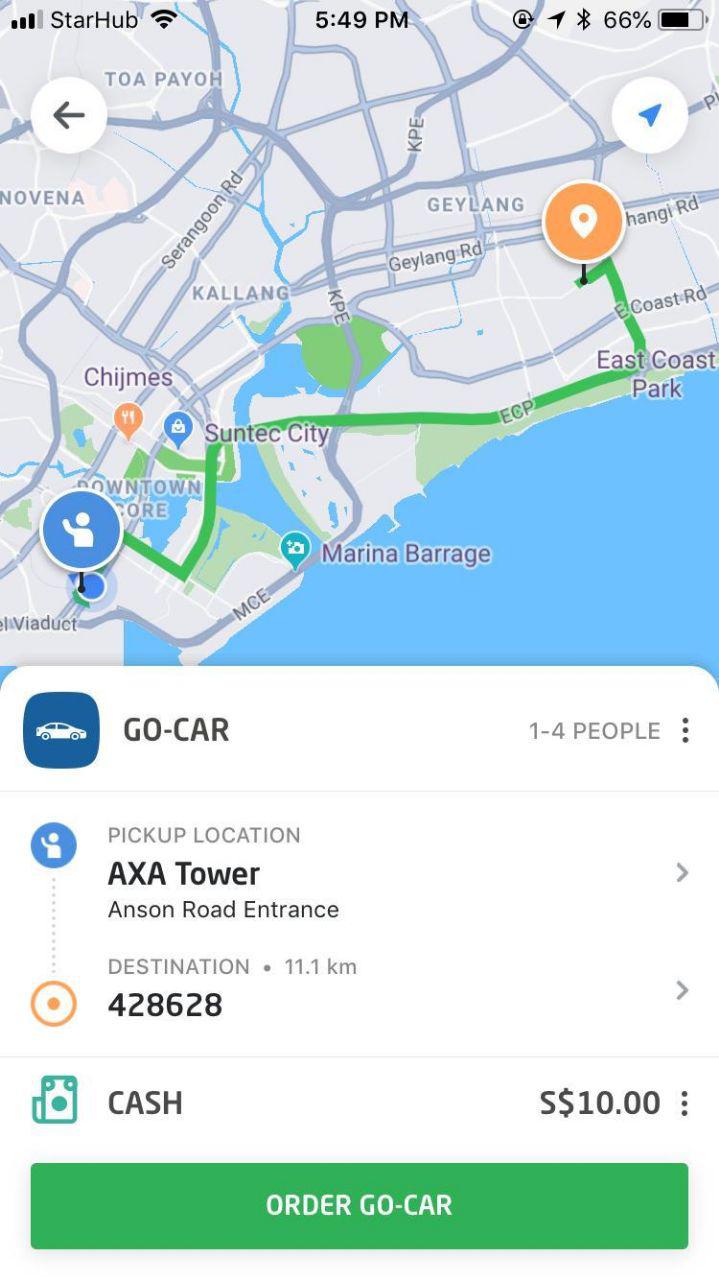A comprehensive screenshot of a map application displayed on a smartphone screen. At the top of the phone's interface, various status indicators are visible: the signal strength shows three out of four bars, labelled "StarHub"; a full Wi-Fi signal icon; the current time displayed as 5:49 PM; a lock icon; a location services icon; an active Bluetooth icon; and a battery icon indicating 66% charge remaining.

The map presented on the screen highlights several key areas, such as Suntec City, East Coast Park, Marina Barrage, Geylang, Kallang, and Toa Payoh, providing a detailed view of the surrounding region. Directions are being displayed for a transport service titled 'GoCar,' which accommodates one to four passengers.

Specific details of the trip include a pickup location at AXA Tower, located at the Anson Road entrance, and a destination that is 11.1 kilometers away. The fare for this journey is listed as $10 in cash. At the bottom of the screen, there is a prominent green button that enables the user to order a GoCar, making it functionally similar to internationally known services like Uber or Lyft.